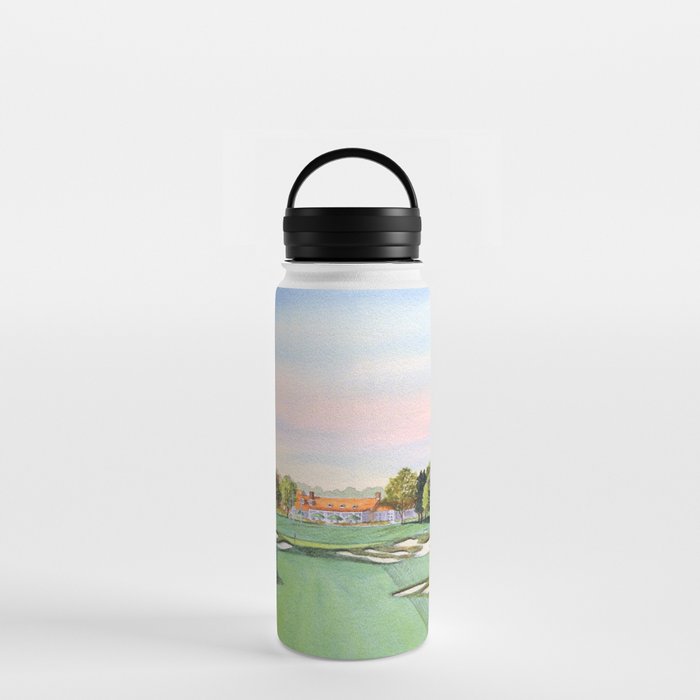This image is a product photograph depicting a white, cylindrical water bottle sitting on a white surface with a pure white background. The bottle features a black plastic screw-on cap equipped with a handle or hoop at the top, allowing it to be easily hung or held. The bottle appears to be wrapped in a detailed watercolor painting, which shows a scenic golf course. The sky in the image transitions from blue to pink, capturing the essence of a pastel-colored sunset. The golf course is finely mowed and adorned with various shades of green grass. Central to the scene is a large, white clubhouse with a distinctive orange, tile roof. Surrounding the clubhouse are green trees with leaves in varying tones, from light to dark green. The water bottle casts a mild shadow to the left, in line with its cylindrical shape. Overall, the photograph makes the bottle appear sturdy and well-made, showcasing a picturesque and serene landscape.